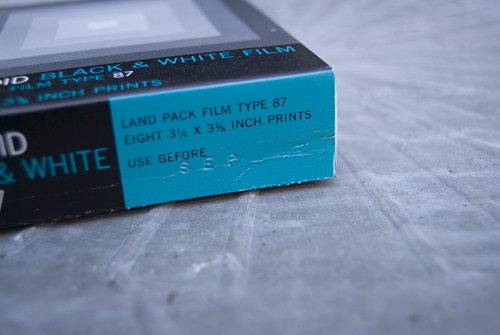The image shows a wide rectangular view of the side of a black box positioned on a textured gray surface with long vertical bumps. The box occupies the top left side of the image, with its edge starting in the middle left and extending outward and upwards to just right of the center. A large turquoise rectangle on the box's edge displays black text reading, "Land Pack Film Type 87, 8 3/4 x 3 3/8 inch prints. Use before." Adjacent to this turquoise rectangle, the black portion of the box features blue and white text that mentions "black and white film" and "film type 87." Above this text is an image of gray concentric squares that gradually darken.